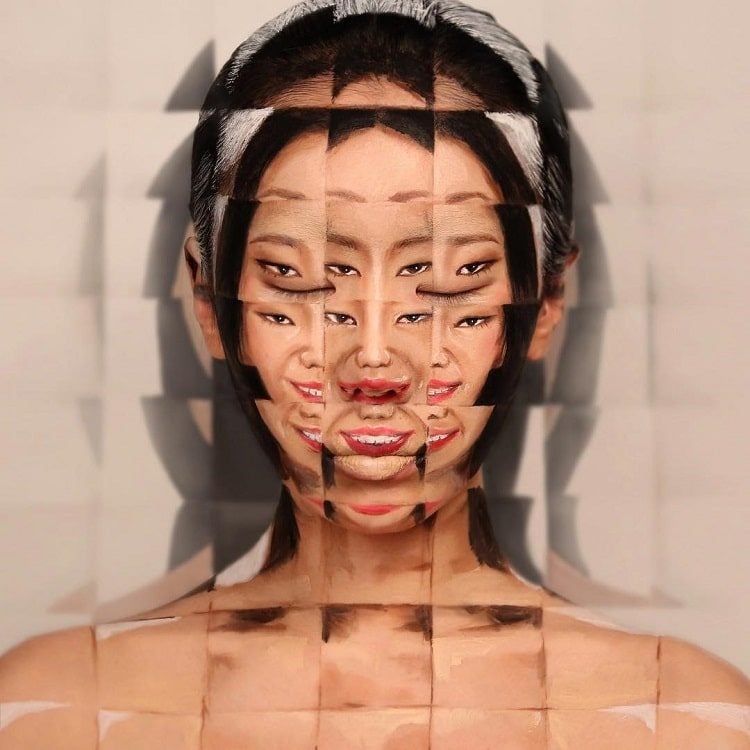This artwork is a composite image of an Asian woman, depicted from her shoulders up. The woman's short dark hair is swept back, and there's a hint of white streaks in it. She has distinct dark eyes, shaped eyebrows, and she is adorned with pink or red lipstick that highlights her smile. Her bare shoulders are visible, accentuating her facial features.

The intriguing aspect of the piece lies in its abstract composition. The original photograph or painting of the woman has been fragmented into numerous overlapping squares. Each square contains a part of her face—a segment of her eyes, mouth, or other facial features—creating a disjointed yet coherent overall image. At the very center is a small version of her face, where she appears without teeth, contrasting with other squares where her mouth displays her teeth.

This artistic effect gives the impression of multiple smaller pictures of her face combining to form a larger, fractured, and complex visage. The woman's expression is enigmatic, with a subtle, sly look that adds to the mysterious and slightly eerie quality of the artwork. This intricate composition makes the image both captivating and unsettling, inviting viewers to delve into its fragmented beauty.